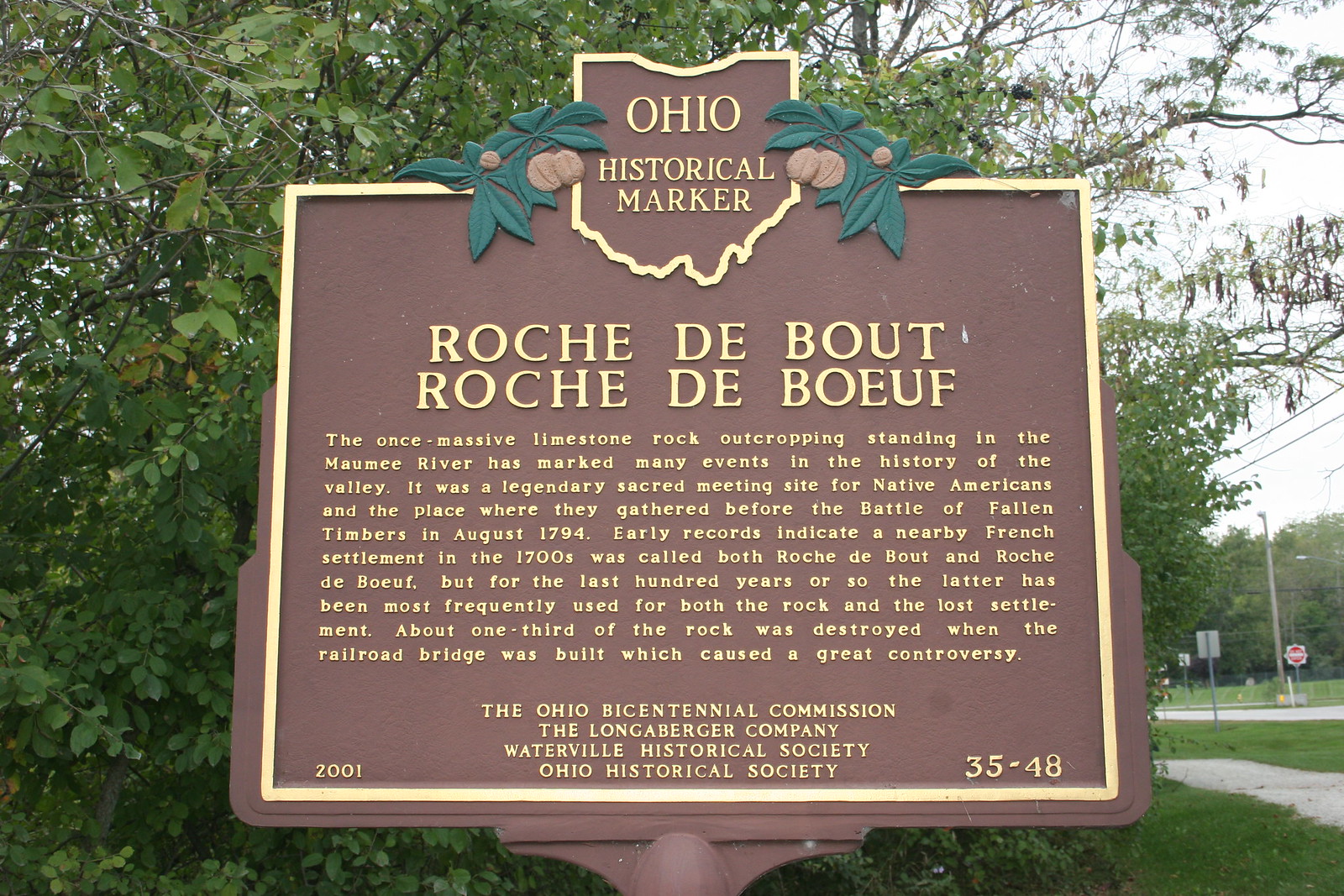The image depicts a brown metal plaque on a post situated on the edge of a road in front of lush green foliage, beneath an overcast sky. In the background to the right, a highway and a sidewalk are visible, along with some road signs and a streetlight. The plaque, adorned with decorative elements featuring leaves and nuts, is titled "Ohio Historical Marker" within an outline of the state of Ohio. The text on the plaque provides historical information about the once massive limestone rock outcropping, known as Roche de Bout or Roche de Bouf, which stood in the Maumee River and was a significant site for many events in the valley's history. This site was a legendary sacred meeting place for Native Americans and served as their gathering point before the Battle of Fallen Timbers in August 1794. The plaque also notes that early records from the 1700s indicate a nearby French settlement bearing the same names. However, for the last century, "Roche de Bouf" has been the more commonly used term for both the rock and the lost settlement. The construction of a railroad bridge led to the destruction of about one-third of the rock, stirring significant controversy. At the bottom of the plaque are the affiliations: the Ohio Bicentennial Commission, the Longaberger Company, Waterville Historical Society, Ohio Historical Society, and the identification number 2001-35-48.